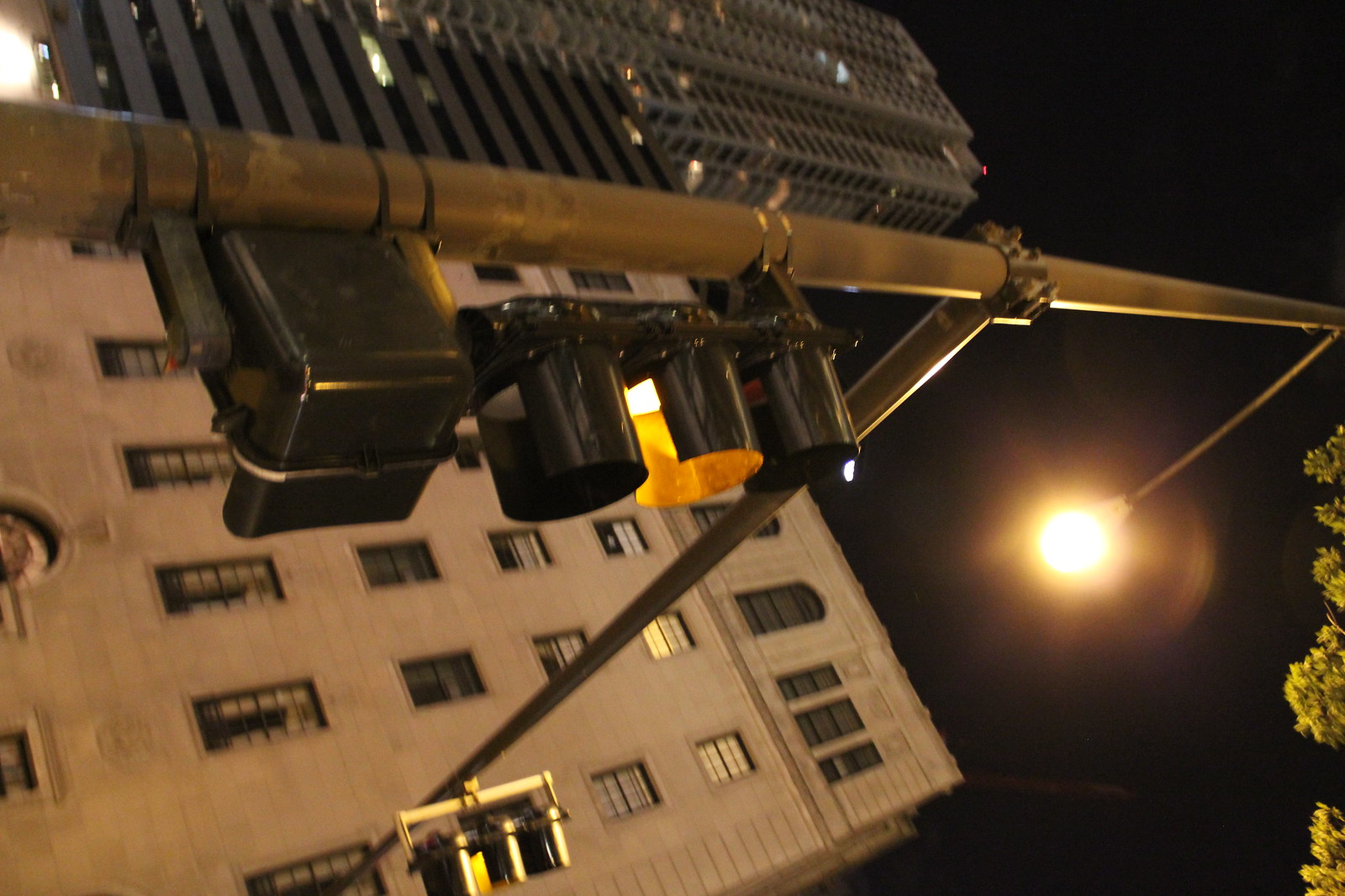The photograph captures a traffic light scene viewed from an unusual angle, almost as if the photographer was lying beneath it. The image, taken at night against a deep black sky, features a gold-colored traffic signal pole running horizontally across the picture, with two traffic lights attached. Both lights, encased in black compartments, show yellow. The main vertical pole also supports a pedestrian signal, although the walk indicator isn't visible. Above the traffic signals, a street lamp illuminates the scene. In the background, a multi-story stone building, partially lit, is accompanied by an even taller skyscraper to its left. The bottom right corner of the image includes a glimpse of green tree leaves.